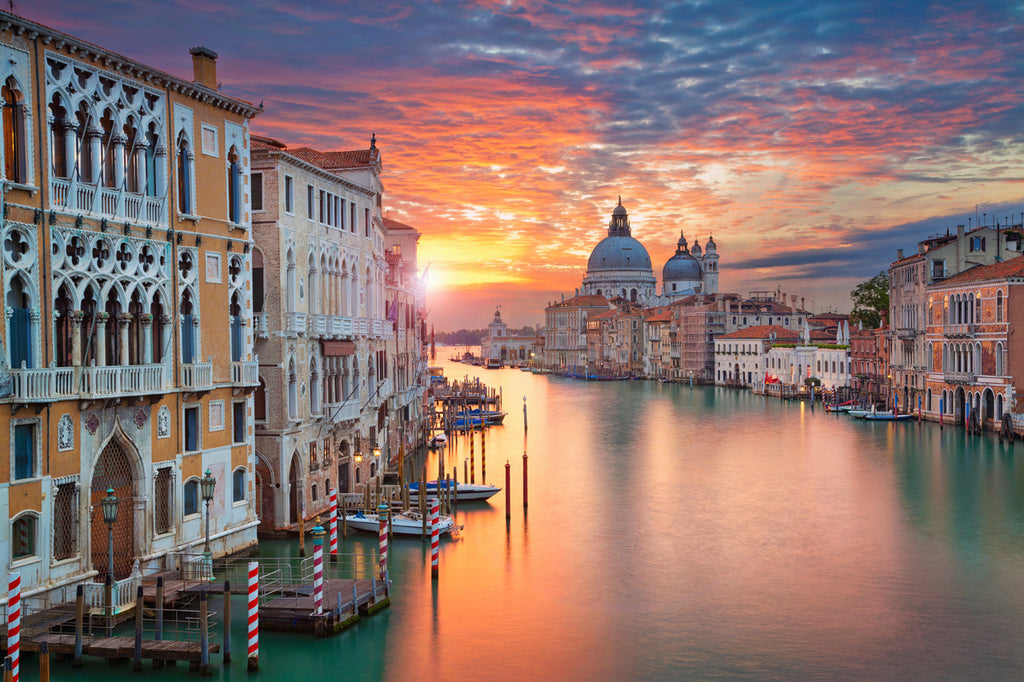This image is likely a painting capturing a serene sundown scene of a canal in Venice, Italy. The canal, which gently curves to the left and then back to the right, is lined with three-story buildings on both sides, creating an almost symmetrical urban landscape. On the left side, a prominent orange building with intricate white fretwork on its balconies stands out, next to a cream-colored structure, both with piers extending into the tranquil water. These piers are adorned with tall, candy cane-striped poles that add a touch of whimsy to the otherwise calm setting. The right side showcases a row of buildings receding toward the vanishing point, where multiple domed structures can be seen in the distant horizon. The canal is dotted with several parked boats, yet the entire scene is notably devoid of people, enhancing the peaceful atmosphere. The water mirrors the stunning sunset, casting hues of orange and gray across the sky, reflected on its glassy surface. This harmonious blend of architectural detail and natural beauty in the sunset, with its orange and purple clouds, creates an almost photographic realism, despite the painterly style.